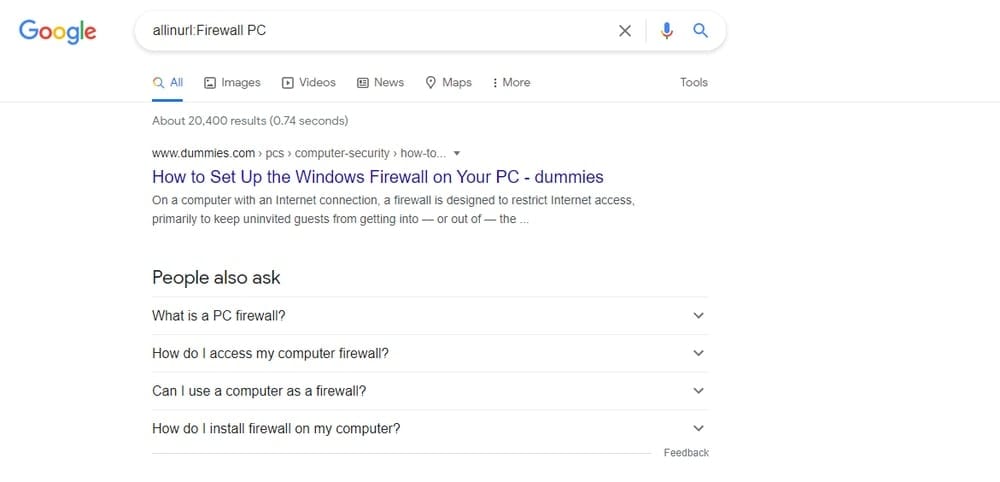The image features a Google search results page. At the top left corner, the familiar Google logo is prominently displayed. To the right of the logo is the search bar, where the query "LE Neural Firewall PC" is entered. Within the search bar, we can also see the 'X' icon for clearing the text, the microphone icon for voice search, and the magnifying glass icon for initiating the search, all aligned on the right side of the bar.

Directly below the search bar, there are six category tabs: "All," "Images," "Videos," "News," "Maps," "More," and all the way to the right, "Tools." The "All" category is currently highlighted in blue, indicating it is the selected tab.

Beneath these tabs, the search results detail the total number of search results available. The first result listed is from www.dummies.com, titled "How to Set Up the Windows Firewall on Your PC-Dummies." Below this result, a "People also ask" section is visible, featuring commonly asked questions related to PC firewalls. The first question listed is "What is a PC firewall?" followed by "How do I access my computer firewall?", "How do I use a computer as a firewall?", and "How do I install firewall on my computer?". Each question is flanked by a right-facing arrow that, when clicked, reveals a common answer. The entire page maintains a clean, white background for easy readability.